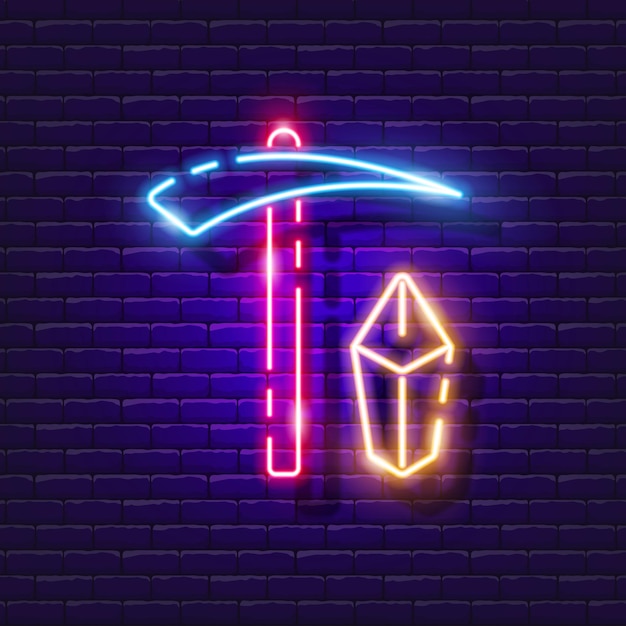The image portrays a dark purple, computer-generated brick wall extending from the bottom to the top of the frame. The wall is adorned with two intricately designed neon signs. On the left, there is a vividly illuminated pickaxe with a red neon handle and a striking blue axe head, characterized by a sharp point facing right. Adjacent to it, on the right, rests a bright yellow-orange neon sign shaped like a box with a triangular top, resembling a gemstone. Both neon signs exhibit a distinctive design style, featuring intentional gaps and floating segments, creating a cohesive and stylistic appearance. The neon lights cast a colorful glow onto the brick wall, enhancing the nighttime atmosphere of the scene.